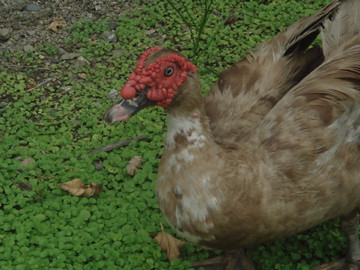The photograph depicts a turkey standing on a flat, green area covered with clover-like leaves and occasional brown dried leaves. The ground also features patches of brown dirt and small rocks, particularly visible in the upper left corner. The turkey, which occupies much of the right half of the image, showcases predominantly brown feathers with hints of white or gray around its neck. Its beak is a combination of pink and black, and it has distinctive red, rubbery-looking skin growths, or caruncles, on its face, typical of turkeys. One noticeable black eye can be seen amidst these red growths. The bird's back feathers are slightly spread open, and it stands firmly on its two orange legs against the vibrant greenery.